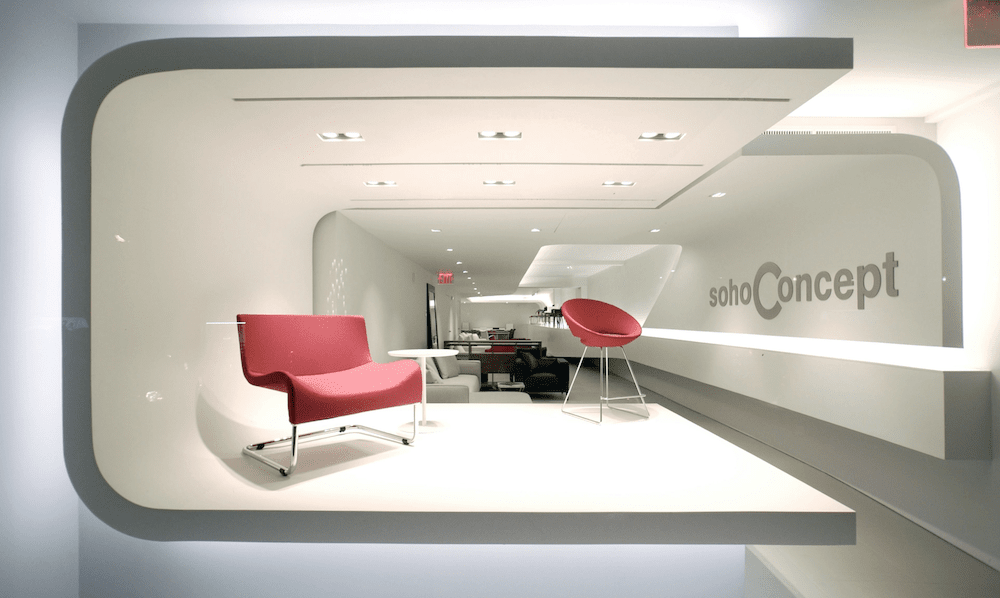The image showcases a narrow, long modern furniture store or conceptual showroom with smooth white or off-white walls, gray trim, and a ceiling lit by spotlights. On the right wall, there's a visible logo in gray letters reading "Soho Concept." The room, resembling a futuristic office or tunnel, has a curved C-shape structure for the left wall, ceiling, and floor. In the foreground, there are two prominent chairs: one, a sleek red chair with metal legs, and the other, a bucket-style chair with a chrome frame and pink leather covering. The background has multiple sofas, couches, and other modern furniture pieces, though due to the perspective, the finer details of these pieces are difficult to discern. The entire aesthetic leans heavily towards modern and possibly avant-garde design, possibly making it an artistic display.